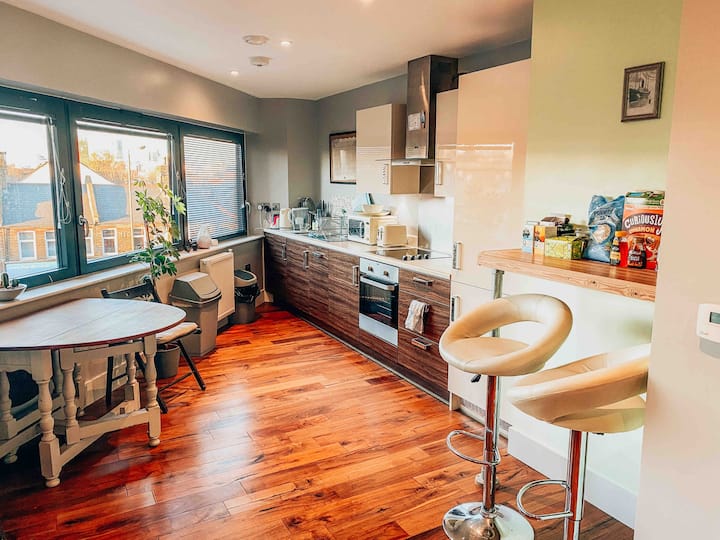This image captures a modern, compact kitchen likely situated in a high-rise condo or apartment, given the visible roofline of a house below, suggesting it's on at least the second story. The kitchen is uniquely shaped with cabinets and appliances arranged diagonally against the back wall, creating an interesting geometric layout. 

The room features three large windows framed in blue, with one of the windows having its blinds drawn. The walls of the kitchen are painted in contrasting colors: a striking green behind a higher bar table, and a darker gray on the remaining walls. The countertops are adorned with various appliances, including a white modern oven, microwave, toaster, and a small fridge and freezer, while the lower kitchen cabinets are stained a dark brown.

A notable feature is a wooden half-table pushed against a white wall, accompanied by a black chair with a cushioned seat. Another focal point is the higher bar table with two white bar stools featuring silver bases and footrests, creating an inviting casual dining area. This table has an assortment of snacks displayed on it, possibly including Cheetos, and above it hangs a small picture of a boat, adding a decorative touch.

In addition, there are two trash cans near the back left corner, assumed to be for regular waste and recycling, placed beside a potted tree plant and a radiator heater. The polished wooden flooring enhances the modern aesthetic of the space, making it cozy and functional.